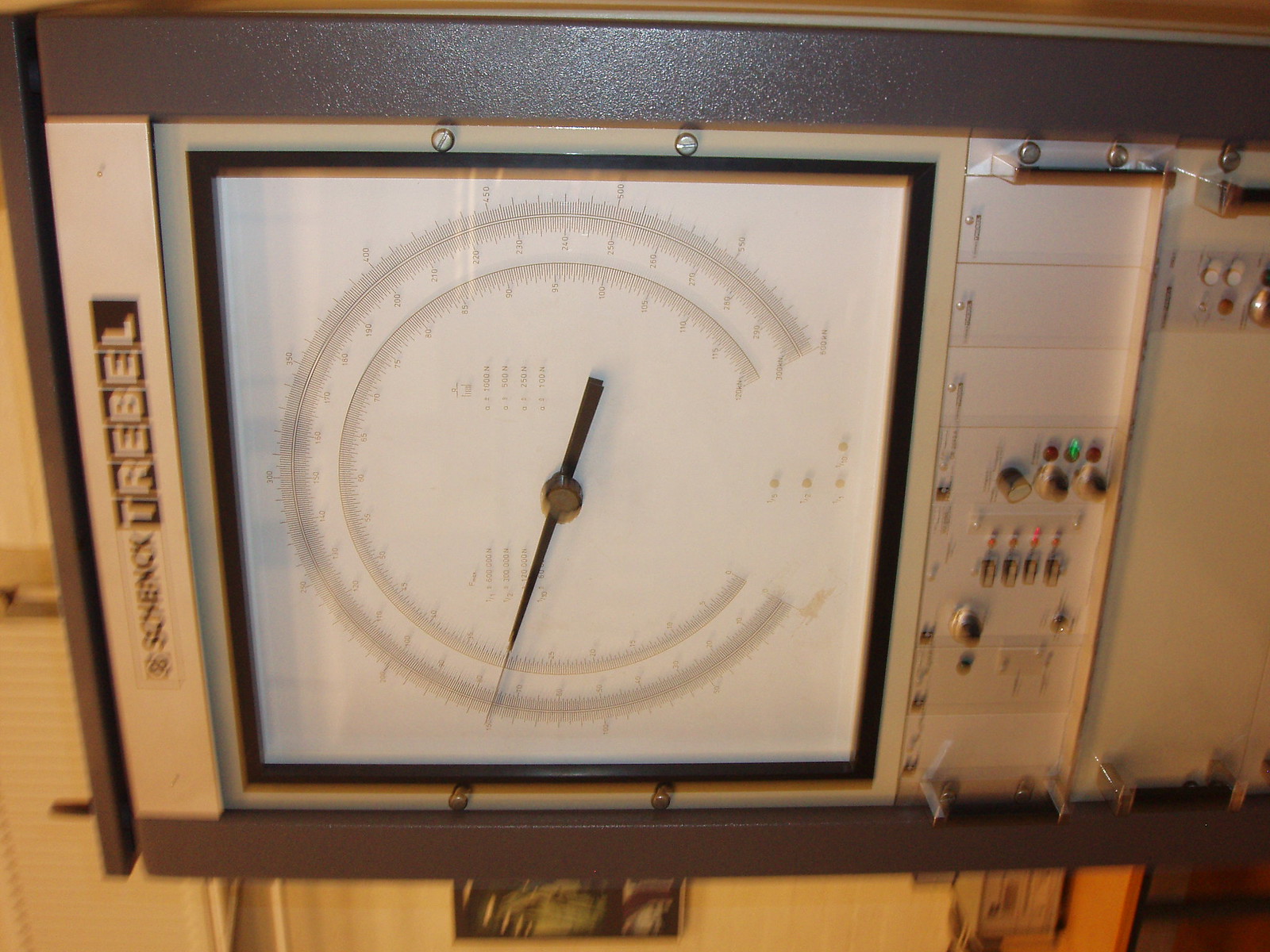The image showcases a utility meter mounted on a light beige-colored wall, which appears to be segmented with a split along the left side. Below the meter, the wall features another split and a hole revealing elements of the electrical works within. The bottom edge of a brown table is visible beneath the meter.

The meter itself is housed in a dark gray box with internal components made of silver metal. On the far right edge of the box, there are metal pieces running across the top, punctuated by small holes and plug-ins. Near this, there is another section of gray metal marked with the number "1" in three sections. Adjacent to this are rows of buttons and indicator lights, which include both green and red lights, followed by a row of switches and an additional black button.

Dominating the center of the meter is a large screen framed by a black border. The screen's face is white, featuring a prominent black hand. Surrounding the hand are numerous small numbers indicating fine increments of measurement. On the side of the meter, a light brown section is labeled "treble."